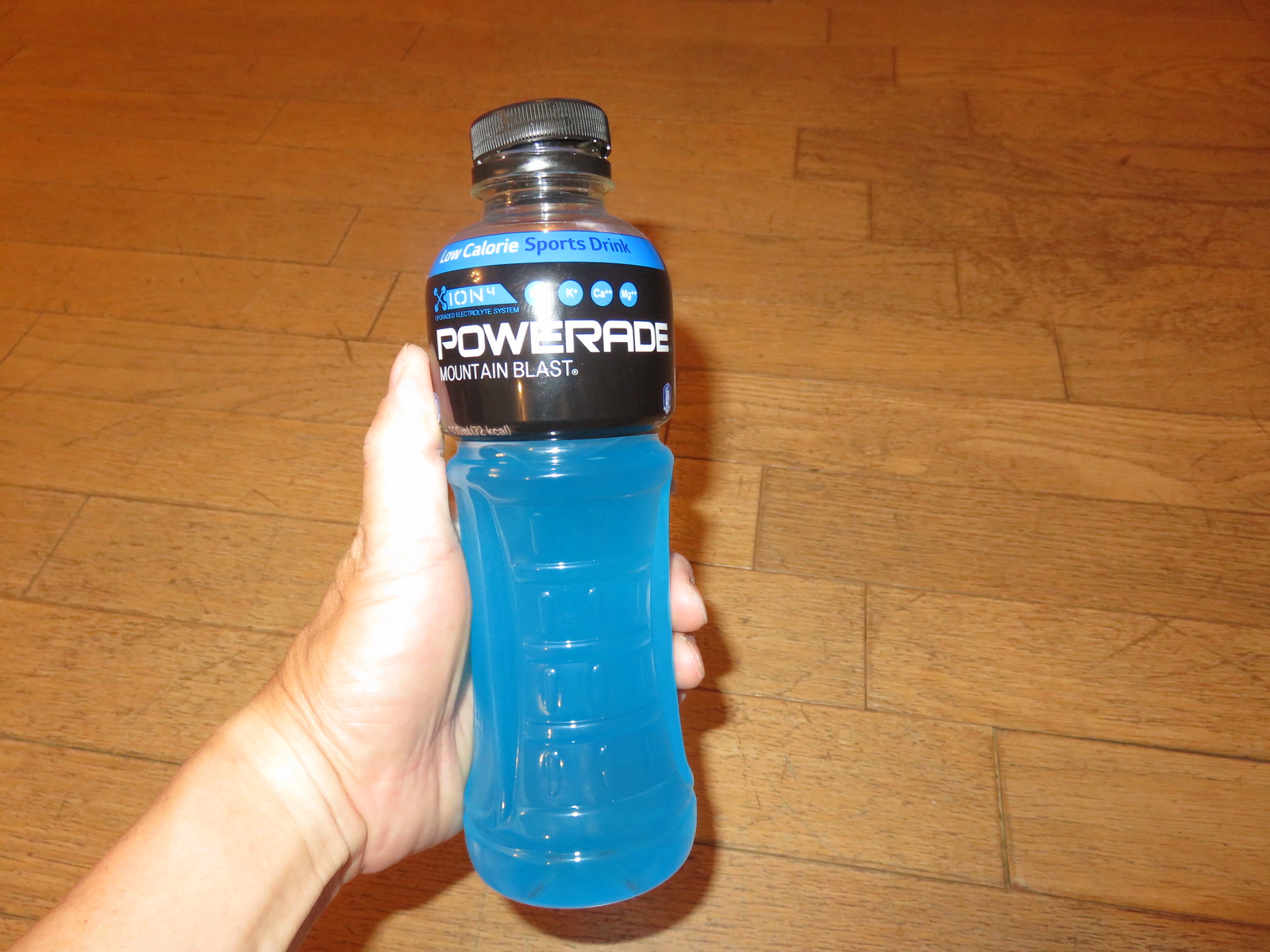In the image, a person, who appears to be Caucasian, is holding a bottle of Powerade over a medium brown wooden floor that shows noticeable scuffs and scratches on its individual planks. The individual is using their left hand, grasping the bottle such that their thumb rests on the side while two fingers wrap around it. The Powerade bottle features an electric blue liquid and has a slightly loosened black cap, indicating that some of the beverage has already been consumed. The bottle's label is predominantly black with white text, displaying "Powerade" prominently along with the flavor "Mountain Blast." At the top of the label, near the neck of the bottle, the text reads "Low-Calorie Sports Drink." Additionally, there are a couple of small blue circles containing white logos and the alphanumeric "ION4" followed by an "X".